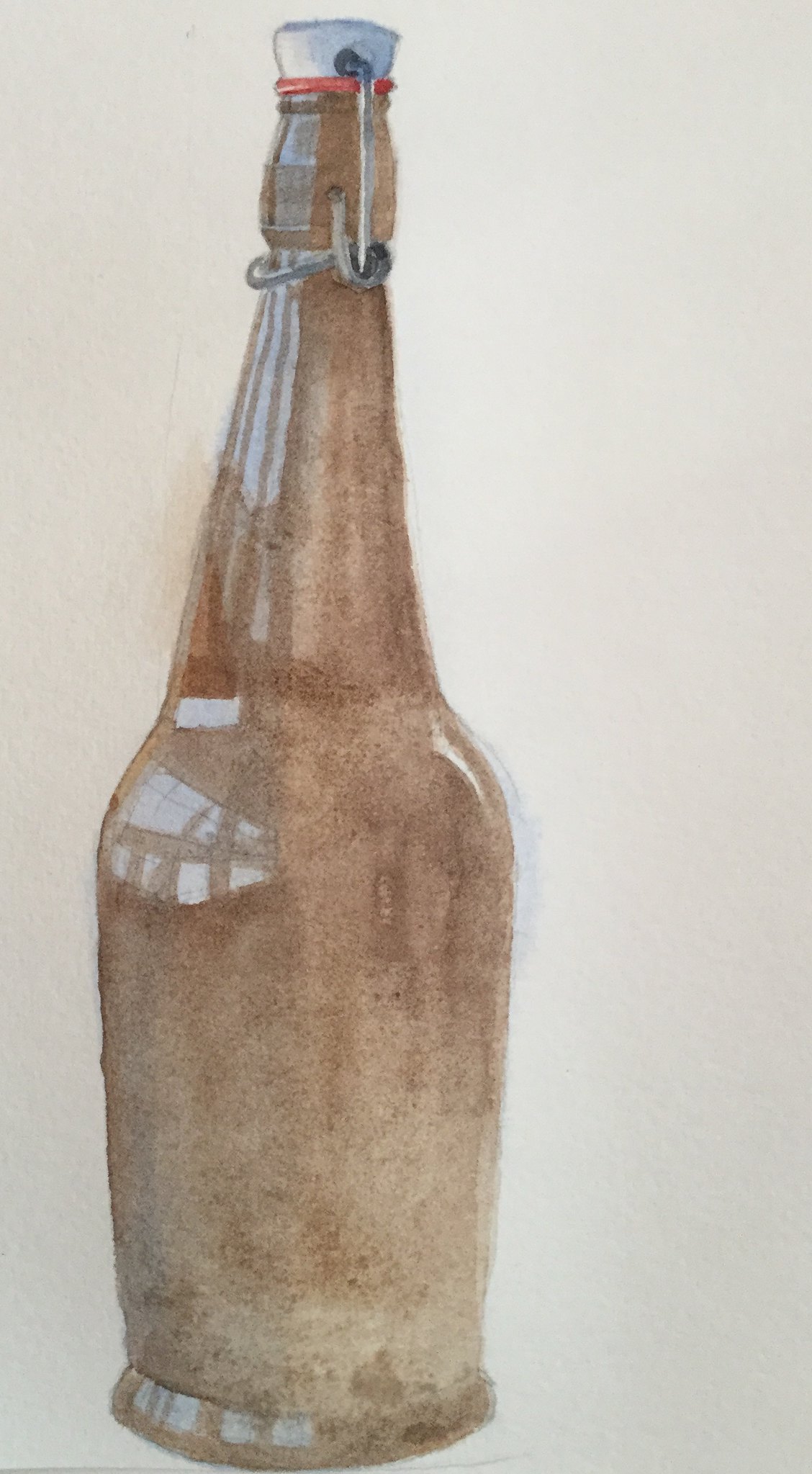This detailed image features an artist's drawing of a tall, slender glass bottle placed against an off-white, textured wall. The depiction is slightly askew and positioned a bit left of center, casting a subtle brownish shadow on the background. The bottle is characterized by its brown hues with varying shades of tan and beige, giving it a distinct, multi-tonal appearance. It includes a re-sealable cork at the top, fastened with a clamp device, similar to those used for homemade oils or water bottles. Reflections of windows and natural light are meticulously illustrated on the left side of the bottle, highlighting its glassy texture. Notable details include a red lip at the top and a plastic plug secured with a pin, hinting at its practical use, perhaps for serving water in a restaurant setting.